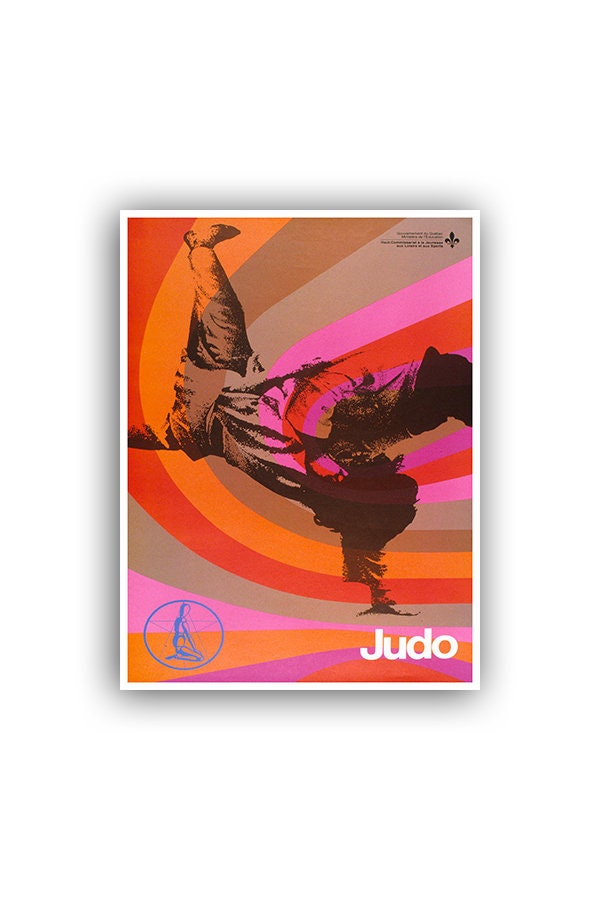The image is a vintage-style poster, likely an advertisement for a judo class, characterized by a distinct rainbow color gradient featuring shades of red, orange, brown, beige, pink, and dark red. At the top right, there's a small black text accompanied by a fleur-de-lis symbol. The central figure in the poster is a man, rendered in a brown hue, who appears to be breakdancing or striking a judo pose, though his face is obscured. At the bottom right, the word "judo" is prominently displayed in white letters. Opposite this, in the bottom left corner, is a circular blue logo depicting a person in a yoga pose, with an indiscernible star design. The overall aesthetic of the poster suggests an era reminiscent of the 1980s or 1990s.